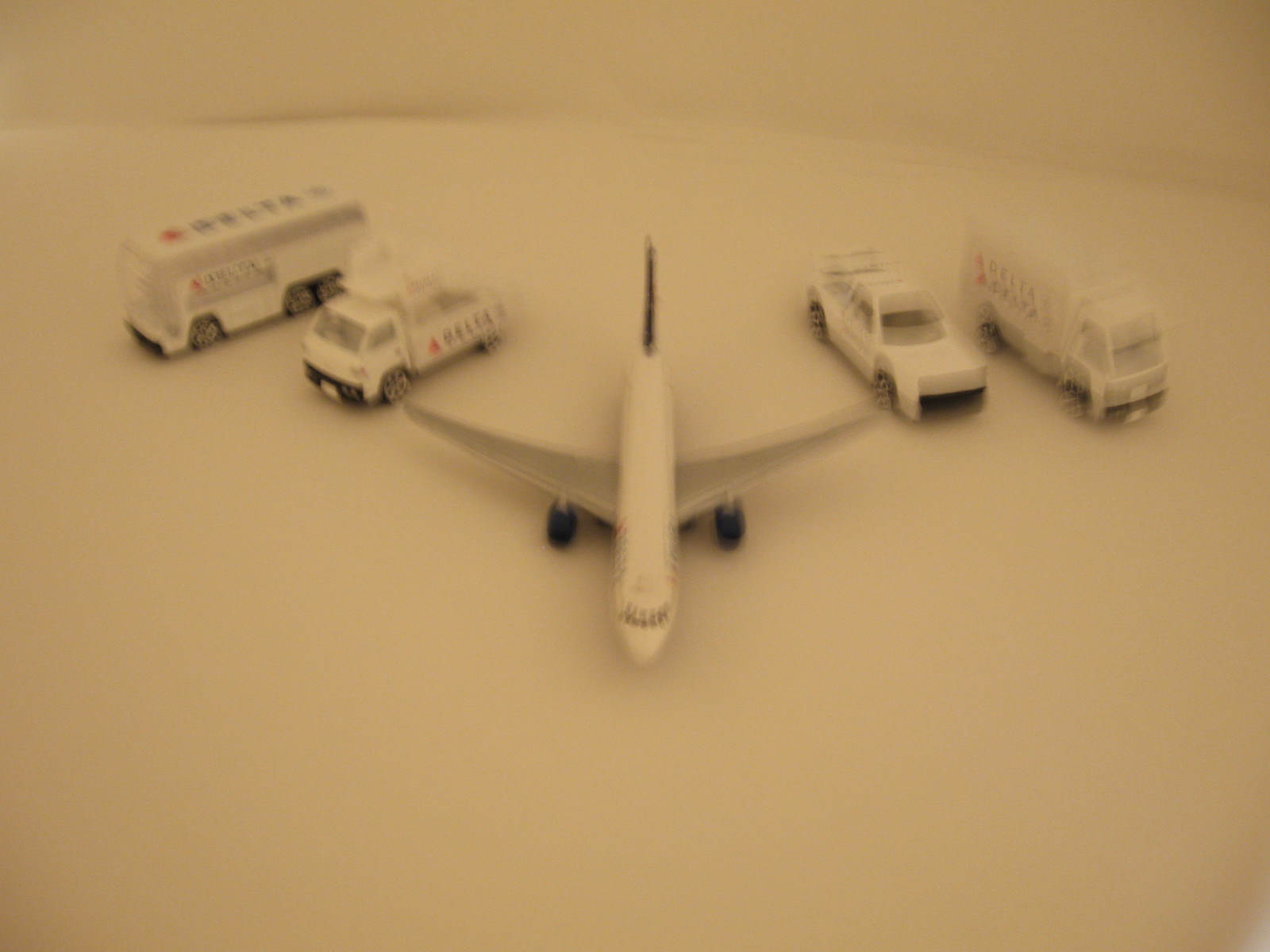This photograph, although extremely blurry, captures a collection of toy models arranged on a surface. At the center of the image is a small commercial airliner model, resembling a Matchbox or Hot Wheels plane, with its wings extending in a distinct boomerang shape. It carries markings indicative of Delta Airlines. To the left of the airplane, arranged in a slightly diagonal V-shape, are a miniature bus and a flatbed luggage carrier truck. On the right side, a white sports car and a large-body cargo van flank the airplane. The entire scene, albeit out of focus, appears to mimic a typical airport runway setup with various airport service vehicles. Hints of white on the ground add to the illusion of a runway environment.